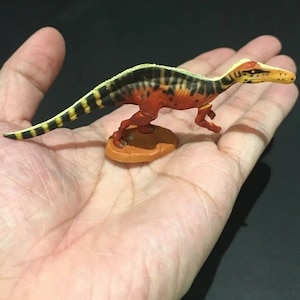In the image, a person's pale white left hand is outstretched, fingers splayed, with a small toy dinosaur resting in their palm. The toy, which fits entirely in the hand, stands on a small orange round base, designed to keep it upright on flat surfaces. The dinosaur itself vaguely resembles a velociraptor and features a detailed color scheme: a yellow and black striped back and tail, an orange underbelly, and a mostly yellow face with black polka dots. The yellow head is notably extended and pointy. The setting has a dark background, possibly black or dark grey, which contrasts sharply with the pale hand and highlights the toy dinosaur and its intricate details, giving the scene a slightly dramatic effect.